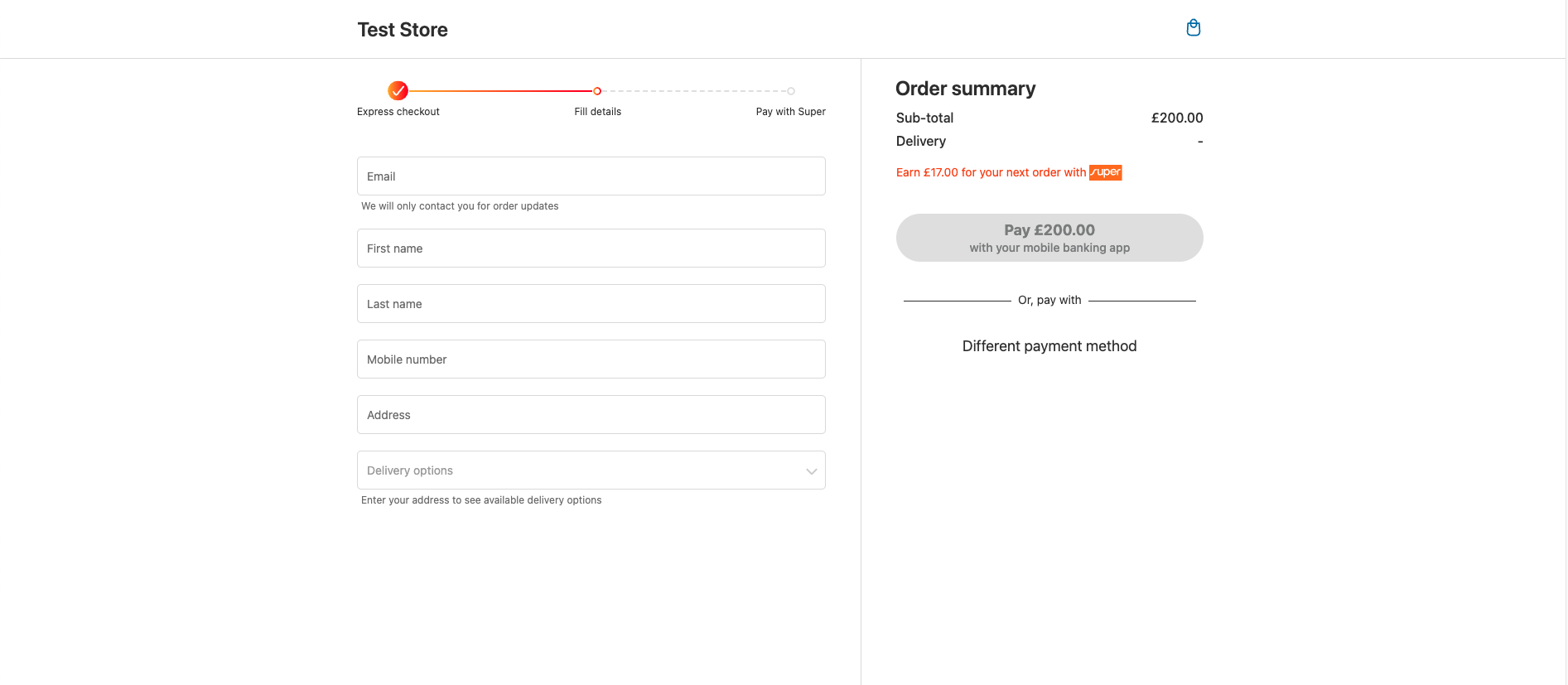This image depicts a user interface for an e-commerce checkout process. At the top of the screen, there is a label that reads "Test Door," accompanied by a shopping bag icon to the right. A horizontal line runs across the width of the layout, beneath the "Test Door" label.

Below this line, a red circle containing a checkmark is prominently displayed. Extending from this circle, a red line travels horizontally to the right, connecting to a segmented grey line. The grey line is labeled with the following steps: "Express Checkout," "Fill Details," and "Pay with Sugar" (assuming the text reads "Sugar").

Underneath these steps, there is a section titled "Email," with a prompt indicating that the provided email address will only be used for order updates. Following this prompt, there are several input fields including: "First Name," "Last Name," "Mobile Number," "Address," and "Delivery Options." An additional note under the "Delivery Options" field instructs users to enter their address to see the available delivery methods.

On the right side of the interface, an "Order Summary" is displayed. This summary outlines the subtotal of £200, with delivery costs left blank. It indicates that users can earn £17 for their next order through some specified means. Finally, a prominently placed button at the bottom of the screen urges users to "Pay £200 with your mobile banking app."